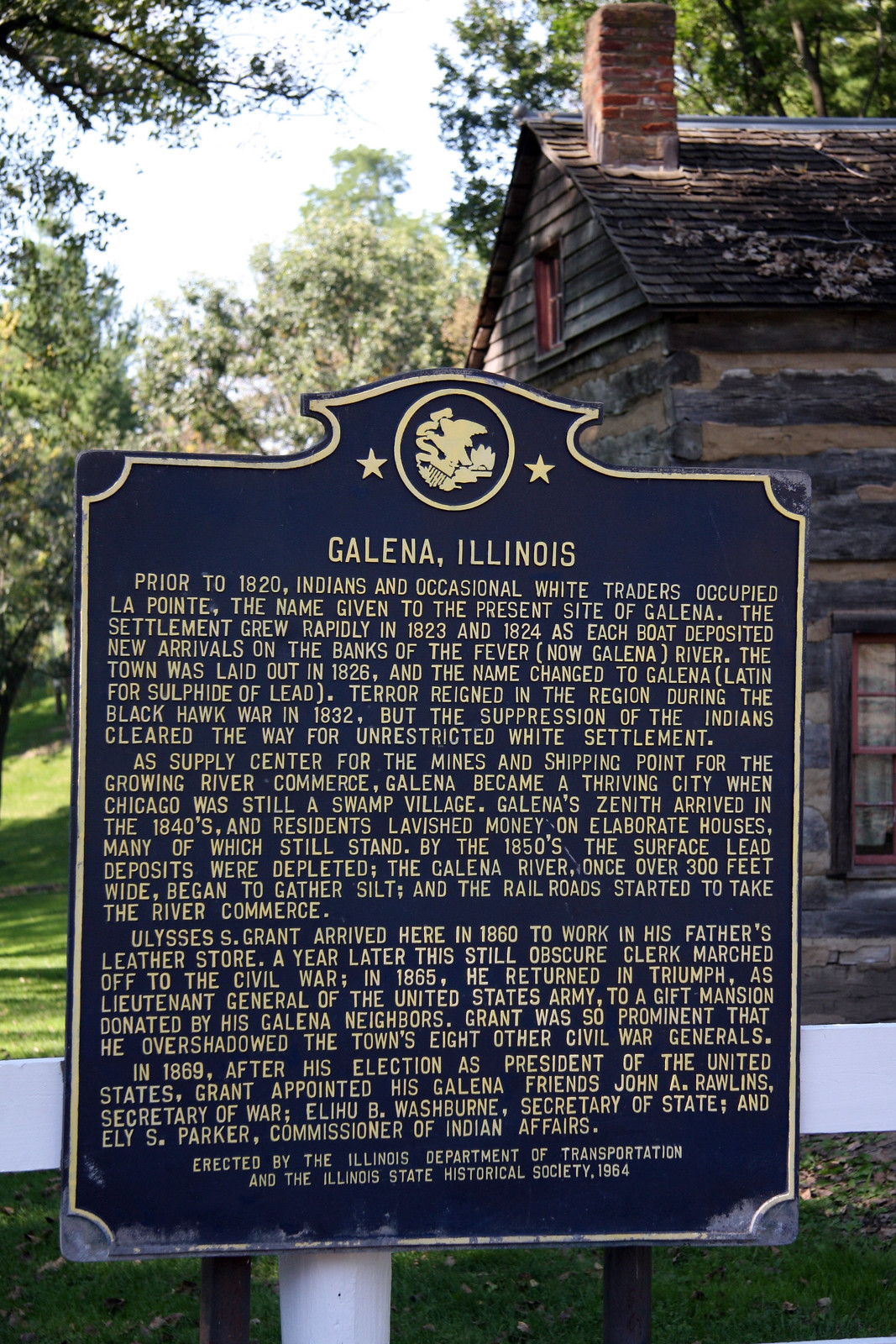This daytime outdoor photograph captures a historical marker stationed in front of a dilapidated old house or cabin, likely made of stone and some wood with a prominent brick chimney. Behind the building, the sky is bright and framed by trees and grass. The blue sign bears a seal at the top and is titled "Galena, Illinois," followed by several paragraphs detailing the area's rich history.

Prior to 1820, Native Americans and occasional white traders inhabited La Pointe, the locale now known as Galena. The settlement expanded swiftly in 1823 and 1824 as boats brought new settlers to the Fever River, currently the Galena River. In 1826, the town was formally laid out and renamed Galena, derived from the Latin term for sulfide of lead. The Black Hawk War in 1832 brought terror to the region, but the subsequent suppression of the Native Americans opened the way for uninhibited white settlement. As a burgeoning supply center for the mines and a shipping point for river commerce, Galena thrived, outpacing many other towns including the then-swamp village of Chicago.

Galena reached its zenith in the 1840s, resulting in the construction of many elaborate homes, several of which still stand today. However, by the 1850s, the superficial lead deposits were exhausted. The once 300-foot-wide Galena River began to gather silt, and the railroad started to eclipse river-based commerce.

A notable historical figure, Ulysses S. Grant, arrived in Galena in 1860 to work in his father's leather store. A year later, he left as an obscure clerk to join the Civil War. Grant returned in 1865 as a celebrated Lieutenant General of the United States Army and was gifted a mansion by his appreciative Galena neighbors. He overshadowed the town's eight other Civil War generals, furthering his prominence. After being elected President in 1869, he appointed several Galena friends to significant positions: John A. Rollins as Secretary of War, Elihu B. Washburn as Secretary of State, and Eli S. Parker as Commissioner of Indian Affairs.

This sign, erected in 1964 by the Illinois Department of Transportation and the Illinois State Historical Society, narrates the prominent history of Galena, Illinois.